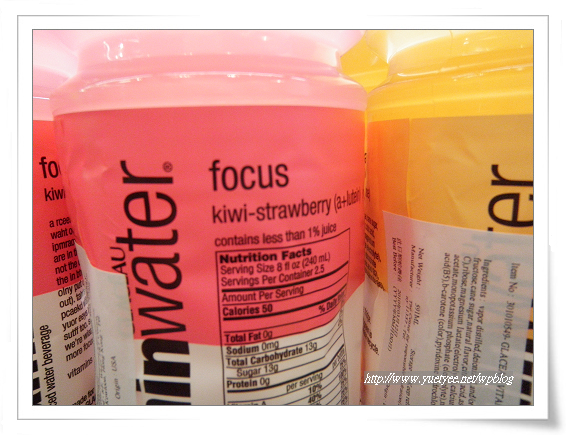The image is slightly rectangular with a horizontal orientation, framed by a thin white border. It presents a very close-up view of two bottles of vitamin water, capturing the middle section up to just before the neck of each bottle. Dominating the scene is a bottle with a pink label prominently marked "Focus Kiwi Strawberry," along with the nutritional facts at the bottom. To its right is the left half of another bottle featuring a yellow label, with the text on this label rendered unreadable. Additionally, just above the labels, the liquids inside both bottles are visible: the Kiwi Strawberry flavor showcases a very pale pink hue, while the adjacent bottle contains a bright yellow liquid.